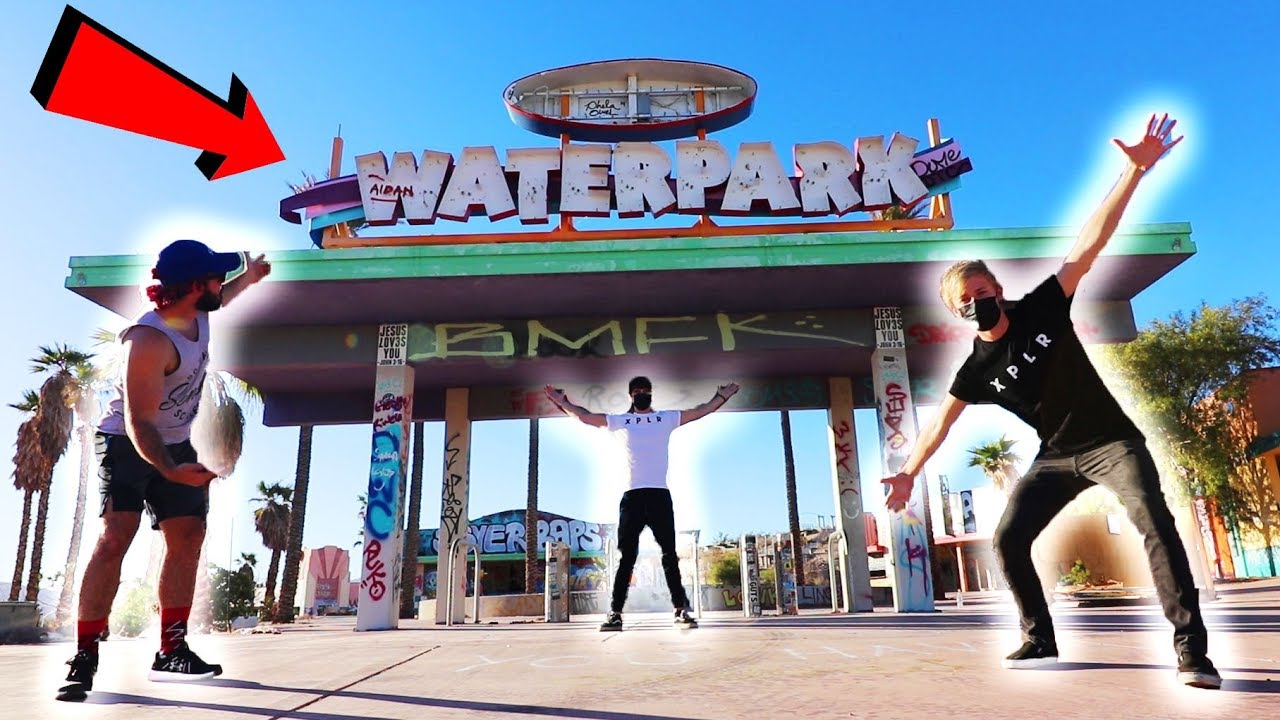This detailed, digitally enhanced full-color photograph captures a clear, sunny day at what appears to be an abandoned water park, suggested by the overgrowth and graffiti-covered surroundings. The horizontally rectangular image features three men, all wearing masks, likely due to COVID-19, positioned in front of a prominently displayed "Water Park" sign at the top center. This sign, framed by pillars adorned with graffiti including the letters "BMFK," is highlighted by a three-dimensional, black-framed red arrow in the upper left corner.

The man in the middle, with his arms outstretched and glowing subtly, wears a white t-shirt emblazoned with "XPLR" and a red bandana over his head. On the right, another man, similarly glowing, stands with his arms extended, dressed in a black "XPLR" shirt and gray Levi denim jeans. The man on the left, turning away from the viewer and pointing up at the "Water Park" sign, wears a gray tank top, gray shorts, a blue cap, and athletic shoes. The scene is backdropped by clear blue skies and tall palm trees, hinting at a California setting.